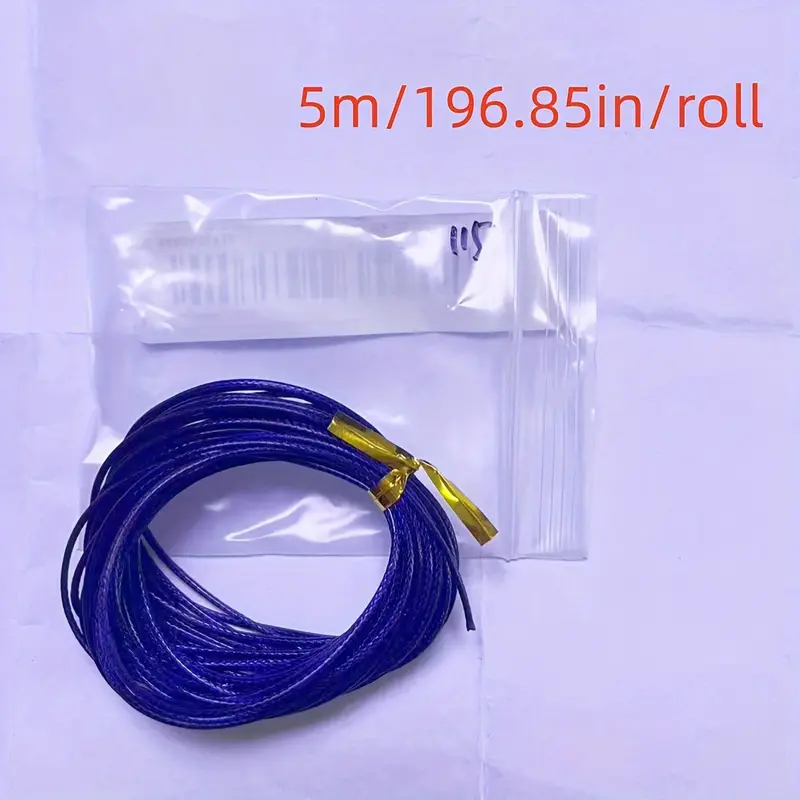This image, taken indoors on a table, features a neatly arranged spool of thin, royal blue, mesh-like wire, coiled and secured with a gold twisty tie. The background consists of a white, folded paper backdrop with red text at the top right corner that reads "5M-196.85IN/ROLL." Just behind the wire, there's a clear, rectangular plastic bag, which likely serves as packaging for the wire. Visible through the plastic bag is a barcode, and an inscription in ink displaying the number "115." All elements combined create an organized and detailed presentation of the product.